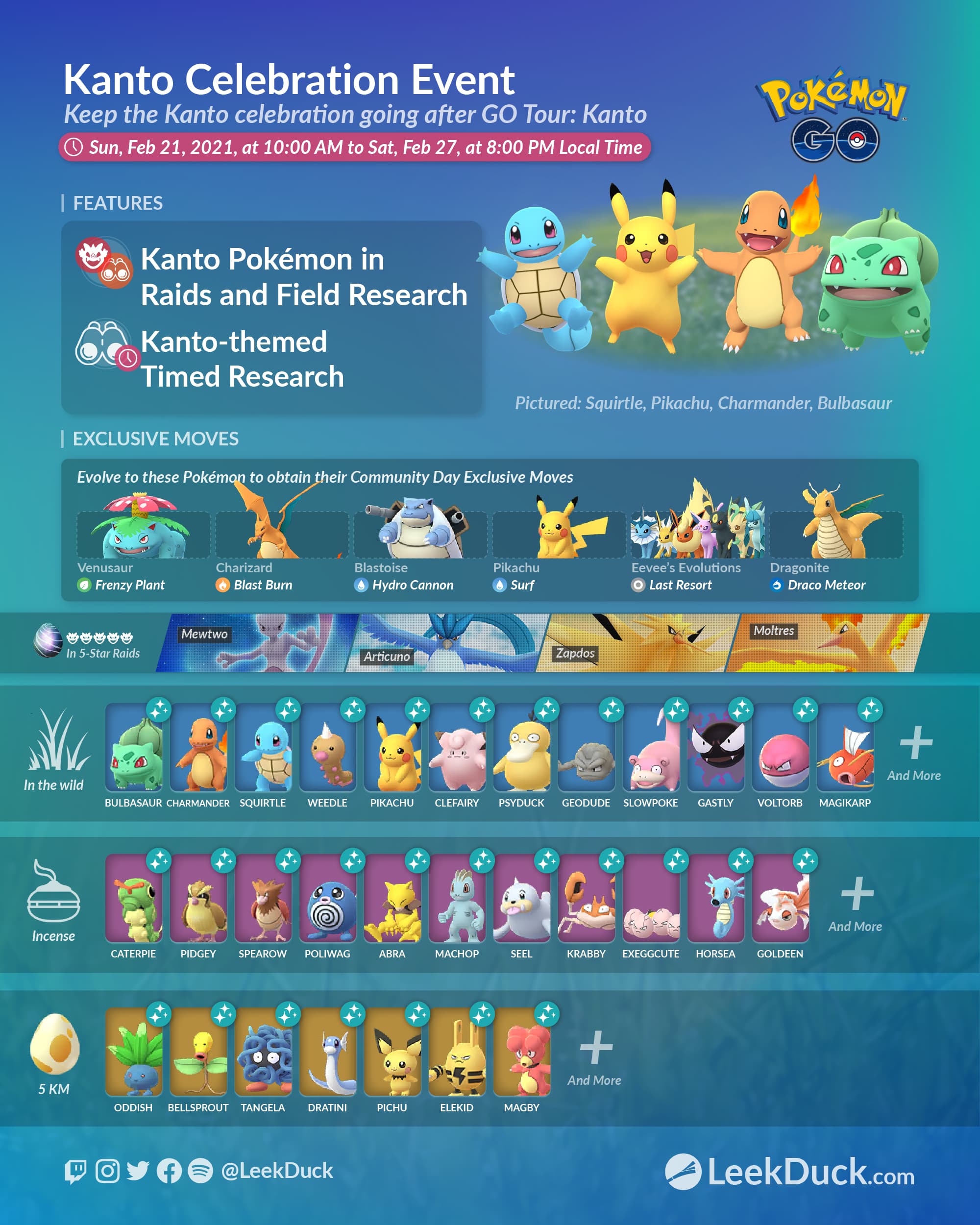Poster Description: 

This is a detailed promotional poster from LeekDuck.com for the "Kanto Celebration Event" in Pokémon Go. The event, designed to continue the festivities of the Go Tour: Kanto, runs from Sunday, February 21st, 2021 at 10 AM until Saturday, February 27th at 8 PM local time. The top section of the poster prominently features iconic Kanto Pokémon such as Squirtle, Pikachu, Charmander, and Bulbasaur as they appear in the game. The poster details various event highlights, including Kanto Pokémon featured in raids and field research, Kanto-themed timed research, and exclusive moves. Additional activities feature Pokémon appearing in the wild, attracted to incense, and available in 5 km eggs. The poster includes images of numerous Generation 1 Pokémon, appealing to fans of the original series, and lists social media links (Twitch, Instagram, Twitter, Facebook, Spotify) in the bottom-left corner for further engagement.